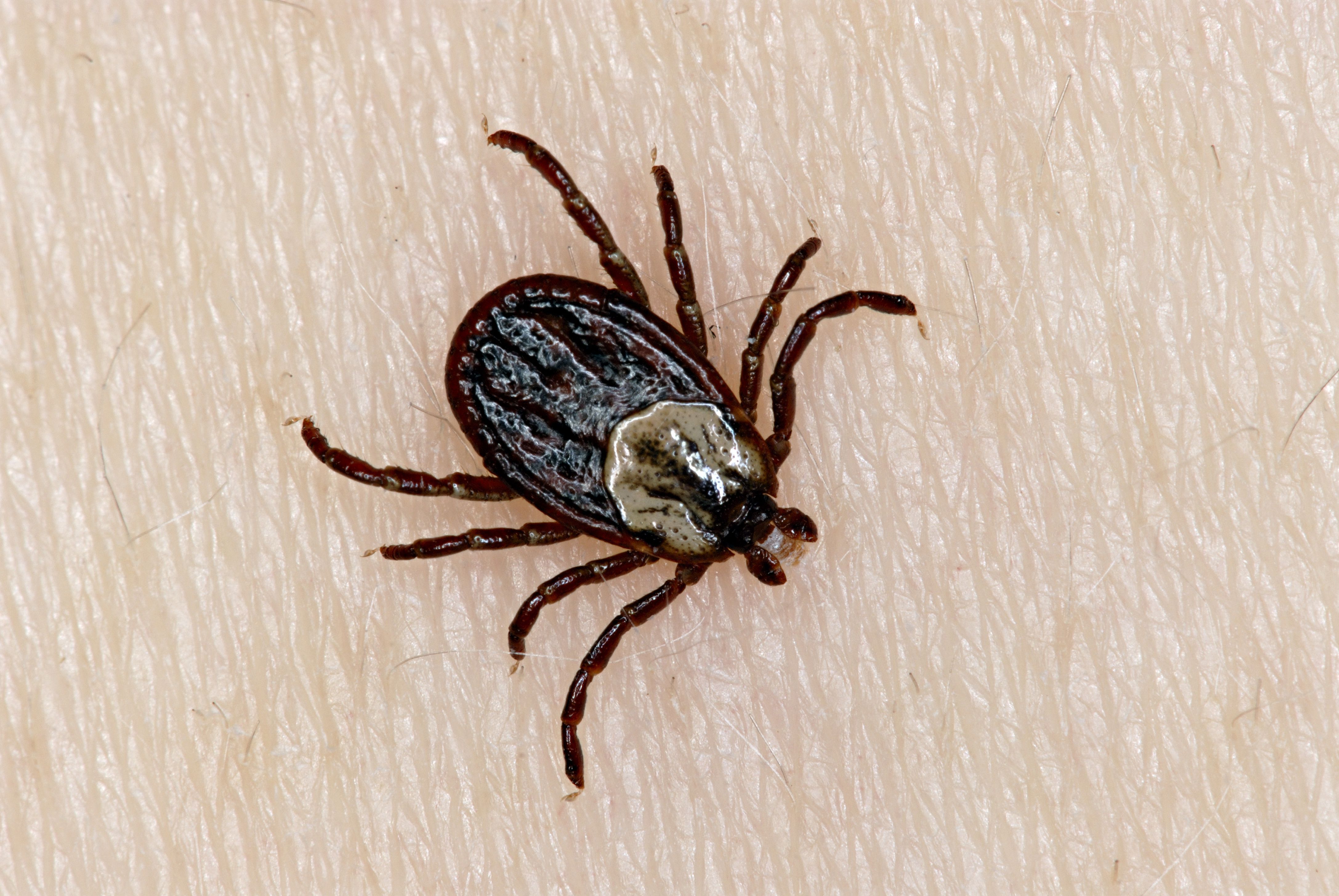A highly magnified photograph captures the intricate details of a small insect, likely a tick, situated on human skin. The extreme close-up reveals the skin's texture with fine hairs protruding, characteristic of an arm. The tick, characterized by its oval shape, boasts eight segmented legs and a dark brown, almost black, crinkled body reminiscent of a raisin. Its head, lighter in color, appears menacing with two notable pinchers. The root beer-like hues blend with subtle beige accents, emphasizing the tick's details against the ruddy surface of the skin.